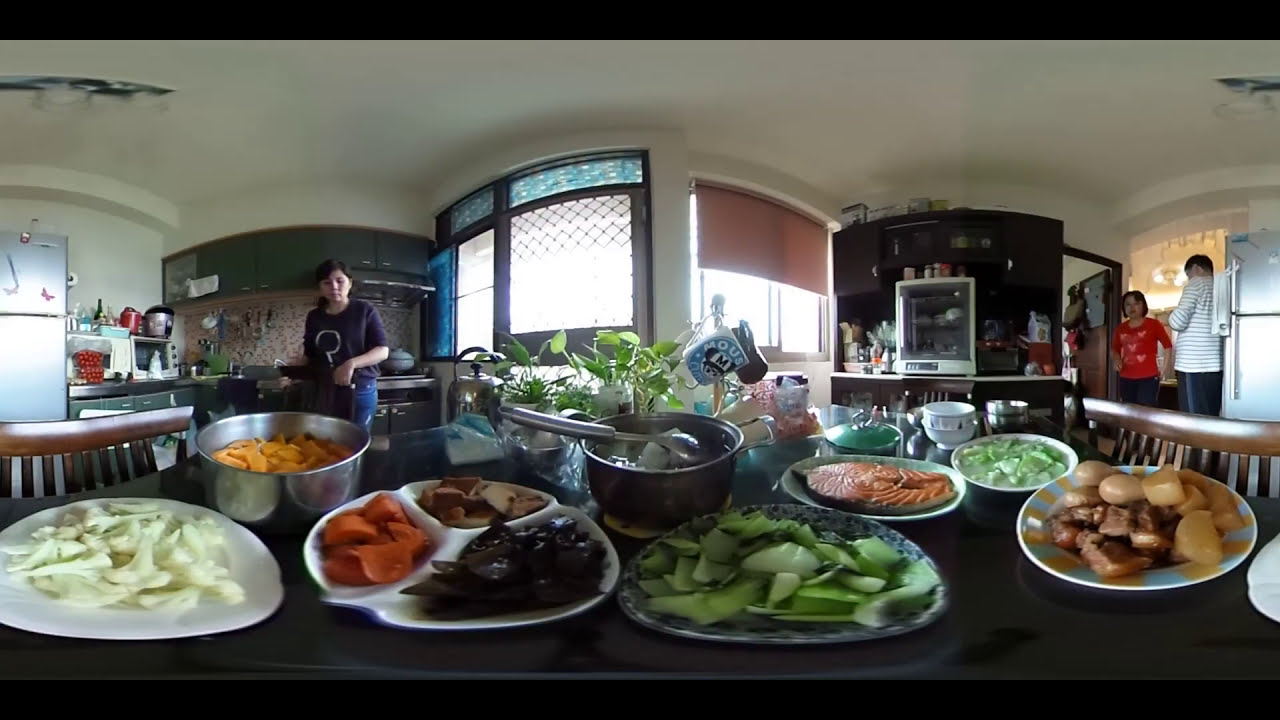The image captures a warm and bustling kitchen scene from a wide-angle perspective, centered on a large black table laden with a vibrant array of foods. The table is surrounded by several brown wooden chairs and features an assortment of plates and dishes, suggesting a gathering or a feast. Prominently, there are vegetables like cauliflower, sliced carrots, and bell peppers, as well as dishes that may include various types of chips, a pot that appears to contain macaroni and cheese, and plates with hummus and green vegetables such as cucumbers.

In the bright and contemporary kitchen, distinct elements include a high white ceiling with hanging lights, pale green cabinets, and a combination of stainless steel appliances. The background shows a curved wall with large windows providing ample natural light. To the right, a stainless steel refrigerator stands out, while another similarly styled fridge is visible on the far left. The left side also has a stove range and countertops hosting several kitchen appliances.

Three people are captured in the frame, enhancing the lively atmosphere. On the right, a woman in a red shirt and jeans stands beside a tall man wearing a white and black striped shirt and black pants, positioned near the right-side refrigerator. On the left, another woman in a black t-shirt with jeans is visible near the counter. The image exudes a sense of preparation and conviviality, likely for a family gathering or a celebratory meal.